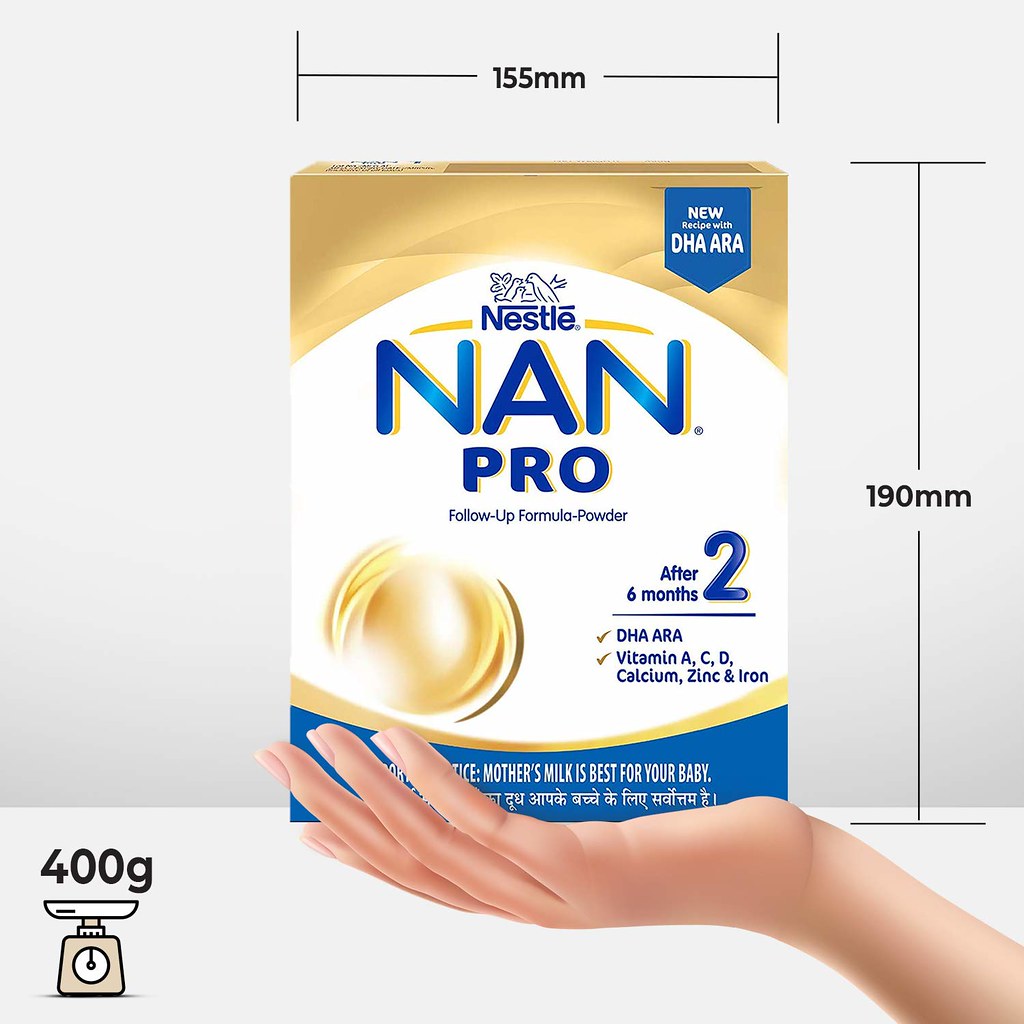This detailed advertisement features a three-dimensional illustration of a box of Nestle Nan Pro, a follow-up formula powder designed for infants after six months. The predominantly gold and blue packaging is topped with a prominent blue label that reads "New Recipe with DHA, ARA." The upper section of the box highlights two key nutritional checks: the first includes DHA and ARA, and the second lists essential vitamins and minerals such as Vitamin A, C, D, Calcium, Zinc, and Iron. Just below the title, the text "After 2, 6 Months" is displayed, indicating its suitability for older infants, followed by more text that says "follow-up formula powder." The bottom left-hand corner of the box indicates a weight of 400G, symbolized by a small line art image of a scale. The advertisement also emphasizes the important notice that "mother's milk is best for your baby," followed by a translation in an Indian language. The dimensions of the box are provided, noting that it is 155mm wide and 190mm tall. The visual is complemented by a graphic hand holding the box, adding a touch of realism to the illustration.